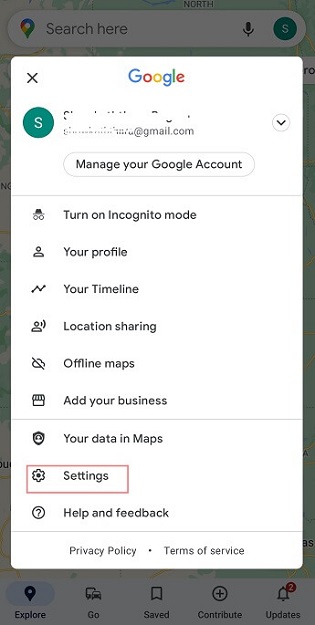The image is a screenshot featuring several key elements displayed within a red rectangle against a very dark, shaded background. In the top section, a microphone icon and the letter 'S' symbolize user control and profile settings respectively. Prominently, a large vertical white rectangle dominates the center, indicating it is a Google interface. At the top-left corner of this rectangle, there is an 'X' icon, and another 'S' icon represents the user's profile. 

Within this interface, the name associated with the Gmail account is visible but obscured by white paint, likely for privacy. A notification bubble that states "Manage your Google Account" sits beside a right-facing arrow. Below, multiple options are listed including: "Turn on Incognito mode", "Your profile", "Your timeline", "Location sharing", "Offline maps", "Add your business", "Your data in Maps", "Settings", "Help", and "Feedback". The "Settings" option is highlighted by a square outline. 

At the bottom of the screenshot, Google's "Privacy policy" and "Terms of service" are noted, aligning with standard service agreements. Additionally, there are icons indicating different functions: "Explore", "Go", "Save", "Contribute", and "Updates".